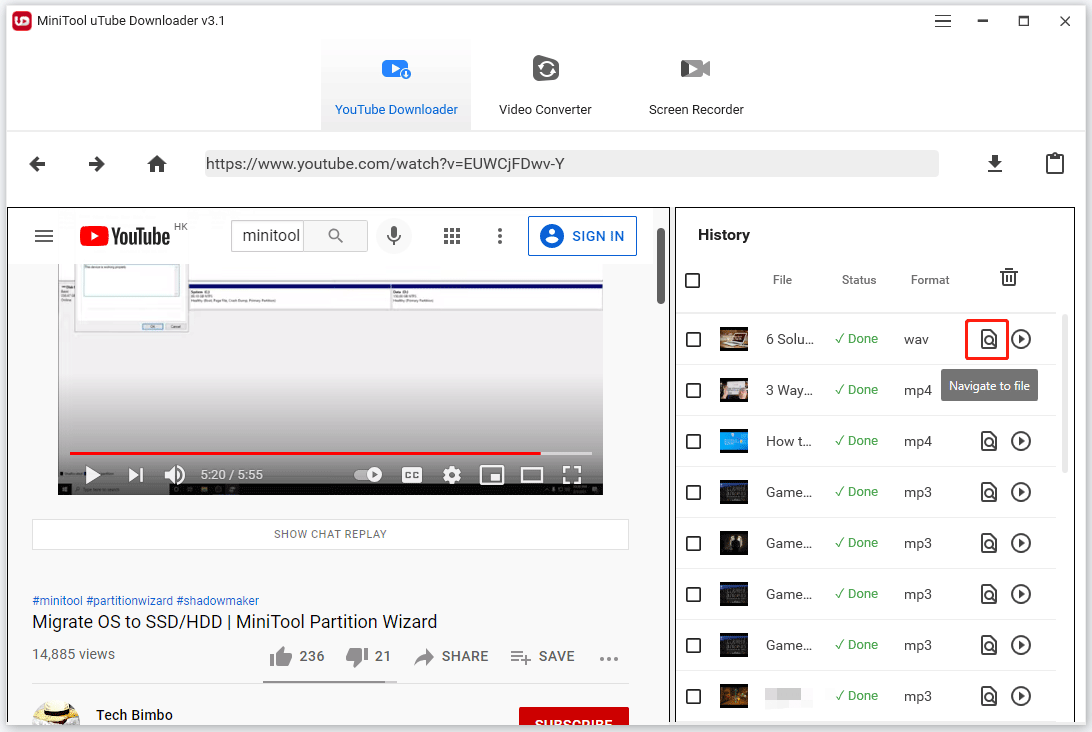This image is a detailed screenshot of the MiniTool YouTube Downloader v3.1 interface. In the top left corner, there is a logo followed by the application's name. The usual window controls for minimizing, maximizing, and closing the application are located at the top right. The main menu at the top center features three options: 'YouTube Downloader' (currently highlighted in blue, indicating its active state), 'Video Converter,' and 'Screen Recorder.'

Below the main menu, there's a navigation bar with left and right arrows, a home button, a YouTube URL input field, a download button, and a clipboard button.

The interface is divided into two primary sections. On the left side, there is an embedded YouTube interface showing a video paused at 5 minutes and 20 seconds into its 5 minutes and 55 seconds duration. The YouTube video player includes standard buttons and features such as the YouTube logo, a search bar, voice control, Google apps, and a blue sign-in button. The shown video is titled "Migrate OS to SSD/HDD MiniTool Partition Wizard," uploaded by the channel 'TechBimbo.' The video has garnered 14,885 views, 236 likes, and 21 dislikes. Under the video, there are hashtags including #MiniTool, #PartitionWizard, and #ShadowMaker, along with options to show the chat replay, a share button, and a red subscribe button.

The right side displays the 'History' section, listing recently downloaded files. Each entry in this list includes a file name (some of which are partially obscured), a status indicated by a green checkmark (signifying completed downloads), a format (with most files in MP3 format except for the top two which are in WAV and MP4), and a trash can icon for deletion. Each file also has an option to navigate to its storage location, represented by an icon of a magnifying glass over a piece of paper.